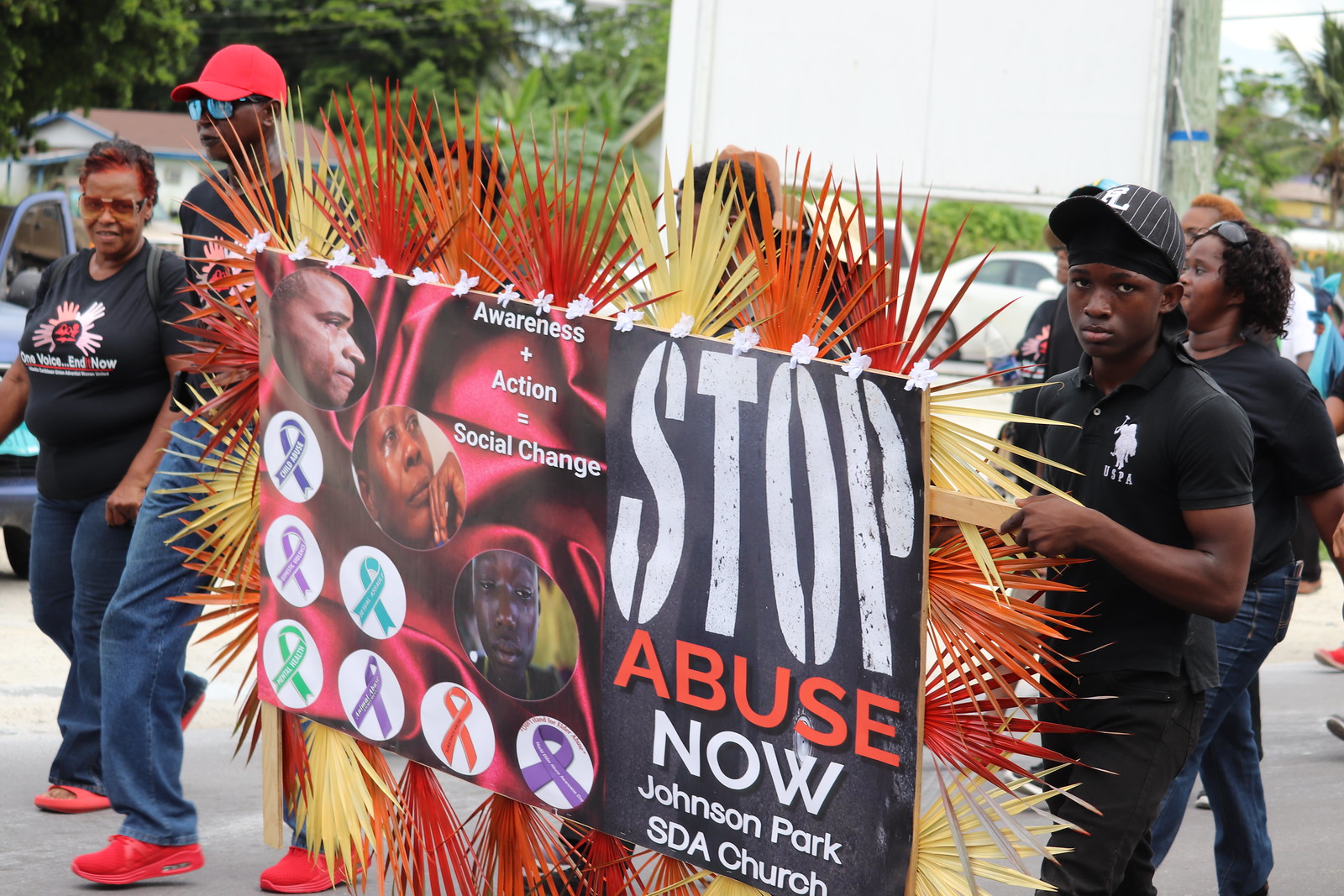In this detailed image of a street parade or protest, a diverse group of African-American individuals is seen marching under daylight. Central to the image is a prominent placard adorned with various symbols and messages. The right side of the placard boldly displays a black strip with the text "Stop Abuse Now, Johnson Park SDA Church," while the left side features the slogan "Awareness + Action = Social Change" against a red velvet background.

Three impactful photographs of African-American individuals dominate the left portion of the placard: an older man with a grim expression, a woman gazing upwards while crying, and another person looking sad and pensive. Below these faces, six colorful ribbons are arranged along the bottom-left corner, though their inscriptions are too small to be legible. The ribbons are colored purple, green, blue, orange, and purple.

Around the edges of the placard, there are decorations resembling feathers or plant fronds. The protestors carrying the placard are clad in black shirts and jeans. Notable among them is a man in his late teens wearing a black USPA polo and a black baseball cap, who stares directly at the camera. Another participant, an older man, is distinguished by his gray mustache, red baseball cap, and jeans.

In the background, additional parade participants and bystanders are partially obscured by the placard and its decorations. Behind them, parked cars, a house, and surrounding trees are visible, underscoring the daytime setting of this poignant and mobilizing event.